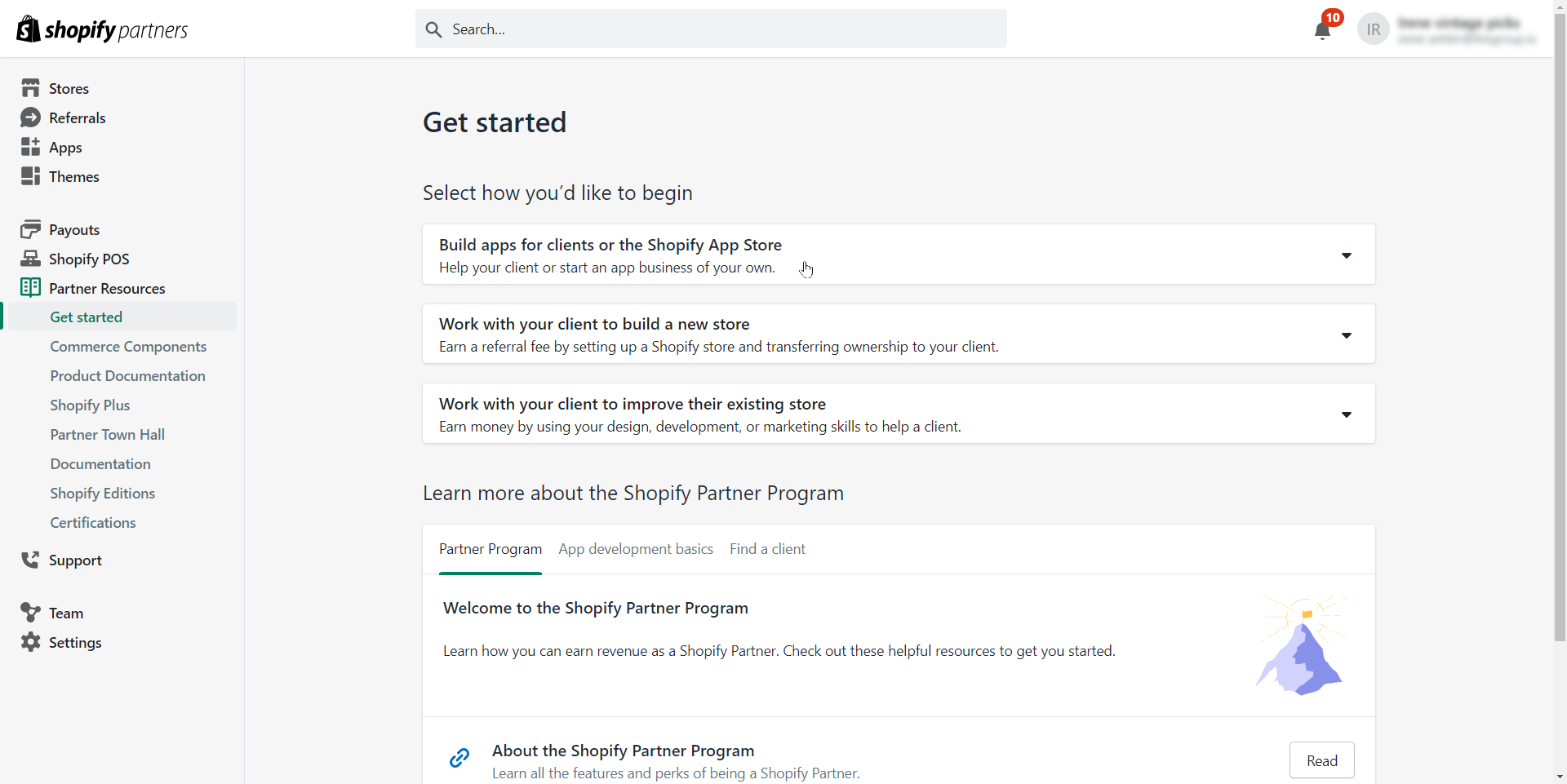This is a detailed and cleaned-up caption for the provided image:

---

The screenshot depicts a logged-in view of the Shopify Partners website. The user's identity is blurred out in the upper right corner, while the Shopify Partners logo is prominently displayed in the upper left. Central to the page is a large search bar. On the left-hand side, a navigation menu lists various sections such as Stores, Referrals, Apps, and Themes. Beneath these, additional options include Payouts, Shopify POS, and Partner Resources, with the latter being selected.

The main content area is focused on the "Get Started" section, which offers multiple pathways for partners. The highlighted text reads "Get Started: Select how you'd like to begin" followed by options such as "Build Apps for Clients or the Shopify App Store," advising partners to help clients or start their own in-app business. The next option is "Work with your client to build a new store," promoting the earning of referral fees by setting up and transferring Shopify stores to clients. Another choice is to "Work with your client to improve their existing store," encouraging the use of design, development, and marketing skills to assist clients for monetary compensation.

Further down, the section offers to "Learn more about the Shopify Partner Program," which is currently selected, revealing a welcoming message: "Welcome to the Shopify Partner Program. Learn how you can earn revenue as a Shopify Partner. Check out these helpful resources to get you started." Below this, a link is provided to "Learn all of the features and perks of being a Shopify Partner," directing users to more detailed information.

Additional support options are visible at the bottom of the navigation menu, including Support, Team, and Settings.

---